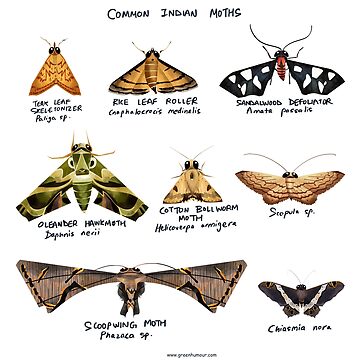This illustrated chart, titled "Common Indian Moths" in a handwritten script style at the top, meticulously showcases eight different types of common Indian moths. Each of the moths is distinctly illustrated, varying in wing size and pattern, with a diverse palette of colors. The intricate designs range from basic beige and brown to striking combinations of green, gold, orange, red, and black. Among the depicted moths are the Teak Leaf Skeletonizer, the Pariga XP, the Rike Leaf Roller, the Sandalwood Defoliator, the Oleander Hawk Moth, the Cotton Ball Worm, the Stopula EP, and the Chiasmia Nora. Notably, one moth features a very long wingspan with black lines and yellow outlines, reminiscent of an upside-down smile in its eye and antenna design. Each moth's name is annotated underneath its corresponding image in the same black handwritten script. At the bottom of the chart, a web URL, www.greenhumor.com, is written in black text.